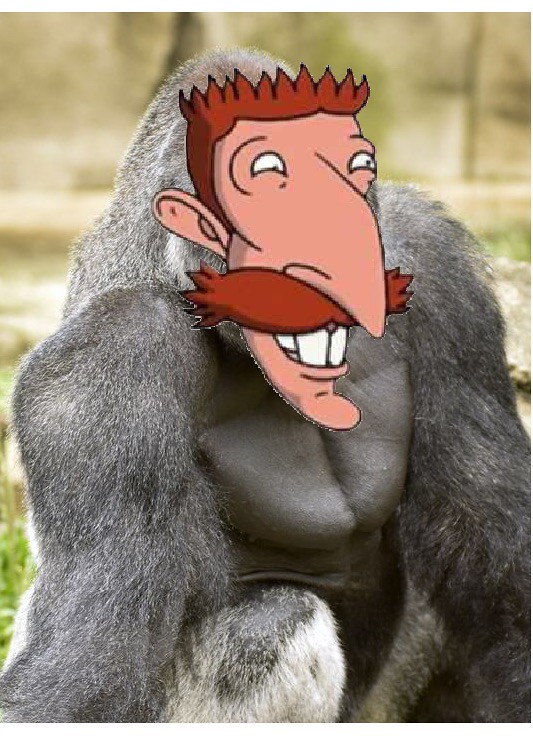In the image, the scene shows a gorilla with a strikingly black and gray fur coat, crouching down with its left knee displaying patches of white. The gorilla's physique is robust, characterized by powerful shoulders and a shiny black chest with sparse fur. The background is a blurry landscape, hinting at green trees and possibly some grass, which contributes to a natural, out-of-focus backdrop.

However, the most distinctive feature of the image is the face. Instead of the gorilla's natural visage, there is a photoshopped cartoon face of Nigel Thornberry from the Wild Thornberrys. This cartoon face stands out with its exaggerated long nose, prominent red mustache, spiky red hair, large ears, and an extended chin. Nigel’s wide smile reveals large teeth, making the image both humorous and surreal. The bright lighting suggests the setting is an open or well-lit enclosure, adding clarity to the strange yet captivating combination.